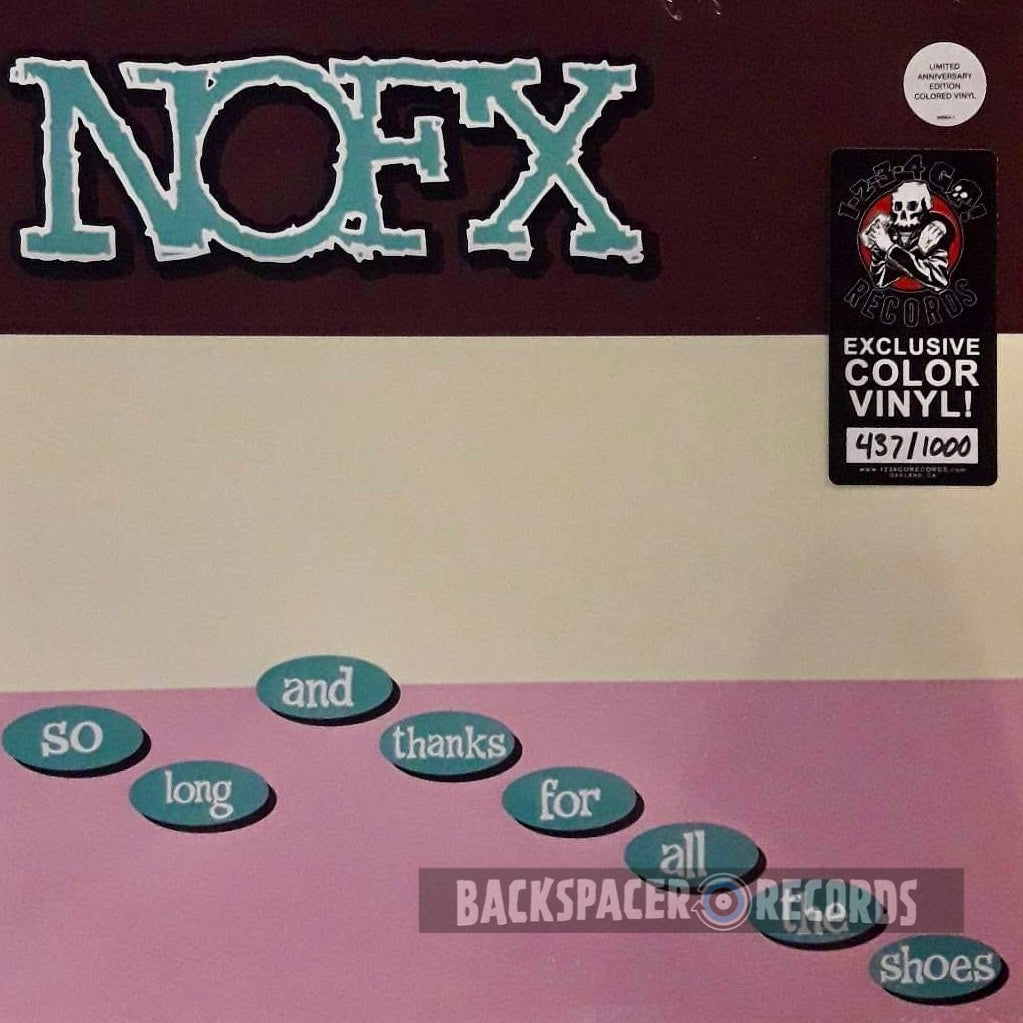This detailed graphic image appears to be a vinyl record cover, arranged in a vertical rectangular layout. The overall background is divided into three distinct color bands: a black band at the top, a beige band in the middle, and a pink band at the bottom. The top black band prominently displays "N-O-F-X" in green letters with a white outline.

In the middle beige section, there is no text or graphic elements. 

The bottom pink band contains multiple green ovals with white writing inside them, spelling out the phrase "So Long and Thanks for All the Shoes." In the bottom right corner, there’s a logo featuring an image of a record flanked by the words "Backspace Records," presumably the name of the label.

Additionally, the top right corner of the cover shows a gray circle with the inscription "Limited Anniversary Edition Colored Vinyl." Underneath this circle is a logo of a person with a skull head and crossed arms, accompanied by the text "Exclusive Colored Vinyl 437/1000," indicating a limited edition release.